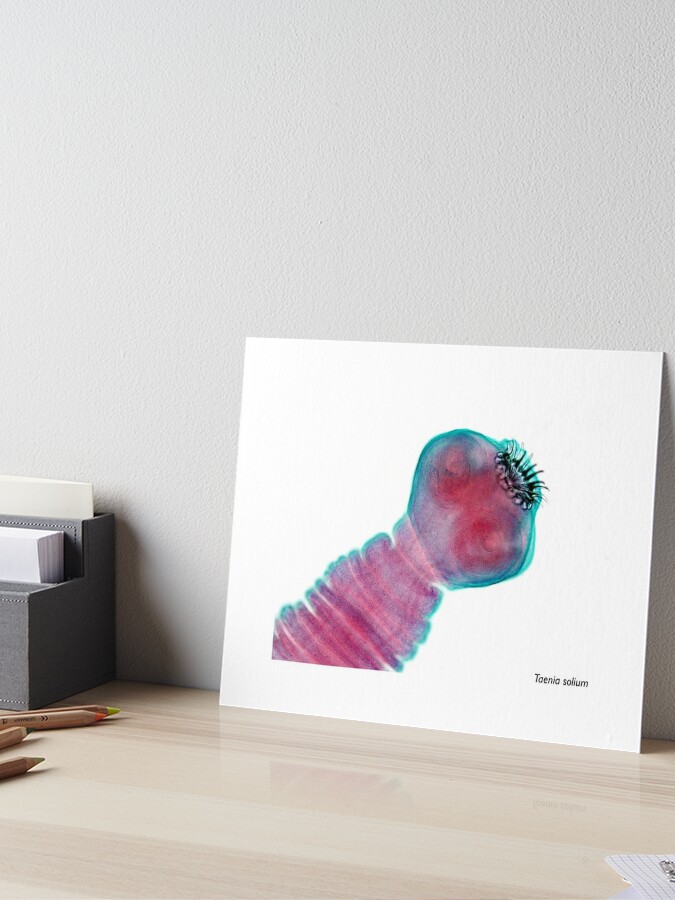The image features a vertically aligned rectangular piece of wall art, resembling a watercolor painting on card stock, leaning against a grey painted wall. The artwork is predominantly white and positioned to the right side of the image. It depicts an abstract, tube-like structure that could either be a vegetable or a sea creature. This structure, starting from the lower left of the artwork, transitions into a furry, circular shape at the top, reminiscent of a mushroom head with seeds emanating from it. The middle section of the tube-like figure is shaded in pink, while the outer edges glow with a bluish hue, possibly suggesting bioluminescence. Towards the lower right corner of the painting, the artist's signature "Tonio Solium" is inscribed in black.

To the left side of the image, there's a grey tray containing a stack of papers, likely index cards, and several colored pencils with wooden brown shafts, their tips slightly visible. The entire setup rests on a desk made of pale brown or beige wood, adding a light and natural contrast to the scene. The setting exudes a creative, artful atmosphere.